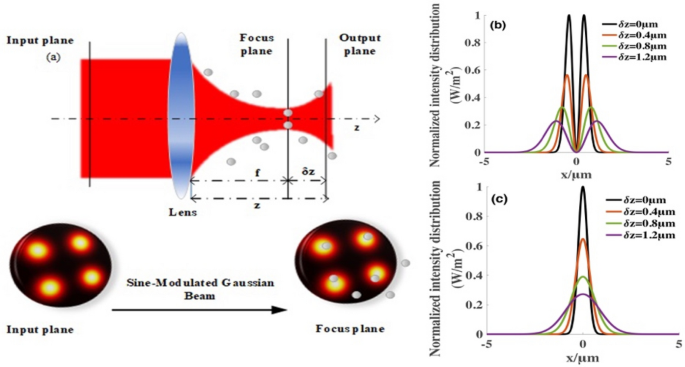This is a highly detailed scientific illustration divided into two main sections. The left side features a red spindle-like object with a blue stripe, described as a lens, passing through three labeled regions: Input Plane, Focus Plane, and Output Plane. The red object narrows at the center, widens again, and includes white dots along its neck area. Below this spindle, there are two black circles each containing four yellow or orange dots, with one labeled Input Plane and the other Focus Plane. An arrow between them indicates the transition as a "Sine Modulated Gaussian Beam." 

The right side showcases two sine wave graphs, one above the other, plotted against an x-axis ranging from -5 to +5. These graphs display peaks at the center with black, red, green, purple, and blue lines, representing different data distributions.